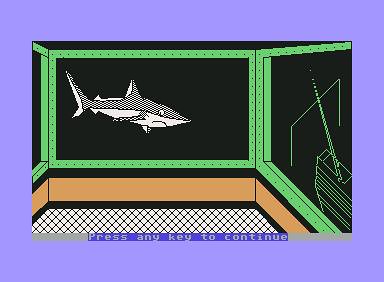This image is a screen capture from a video game, depicting a room equipped with three large monitors. The central monitor features a striking black background with green trim, displaying a black and white image of a shark swimming. Adjacent to this, the monitor on the right presents a different scene, likely a boat, characterized by a mast and crossbeam supported by two vertical poles. Below these screens, the room's interior boasts a checkered floor pattern, complemented by a tan wall adorned with black trim. This detailed setting immerses the viewer in a technologically advanced yet visually compelling environment.